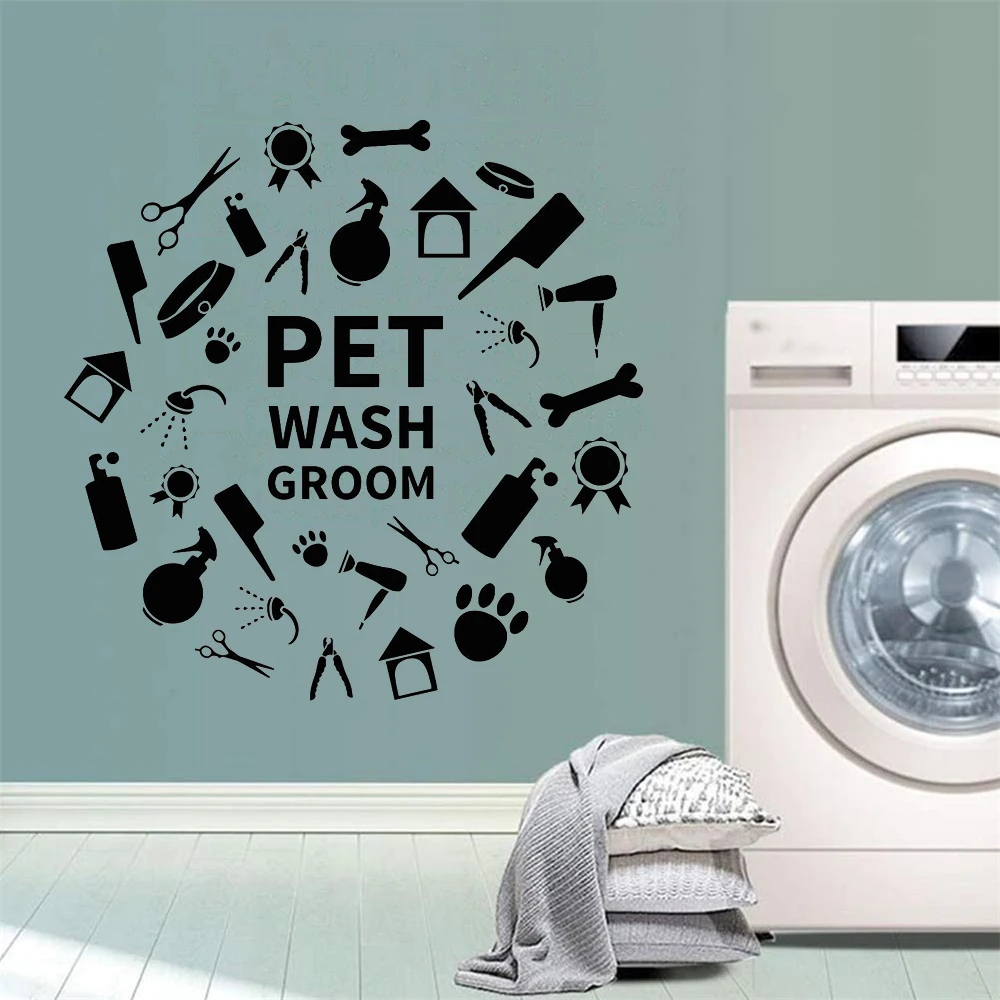The photo captures a room with teal-colored walls adorned with a circular arrangement of various pet grooming icons, including a collar, feeding bowl, plastic bone, pair of scissors, and comb, centering around the words "PET WASHROOM" written in black capital letters. The floor consists of white wooden panels. On the right side of the image, there is a small, front-loading white washing machine, featuring a central door for clothes and a small black control screen on top. To the left of the washing machine lies a stack of three pillows in white and grey hues, with a small grey blanket draped over them. This scene suggests a space dedicated to pet care, specifically grooming and washing.